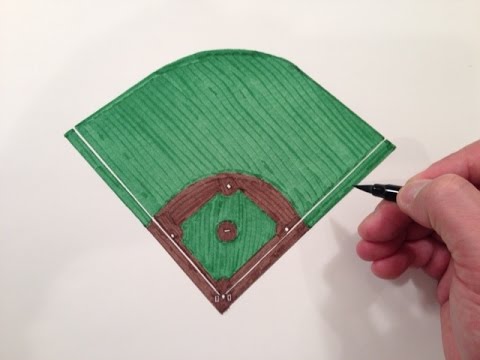The image depicts a detailed drawing of a baseball field on a white piece of paper. The field is illustrated using markers, with the outfield shaded in green and the bases and pitcher's mound marked in brown. The foul lines, drawn in white, extend from home plate to the outfield, clearly delineating the field of play. The paper itself is cut into the shape of a baseball diamond, with a pointed bottom and rounded top. On the right side of the image, a person's pink hand, holding a black-cased marker, is visible, adding a touch of realism to the scene. The intricate details of the drawing, including the brown tracks connecting the bases and the green grass in the outfield, showcase the meticulous effort put into recreating the classic layout of a baseball field.